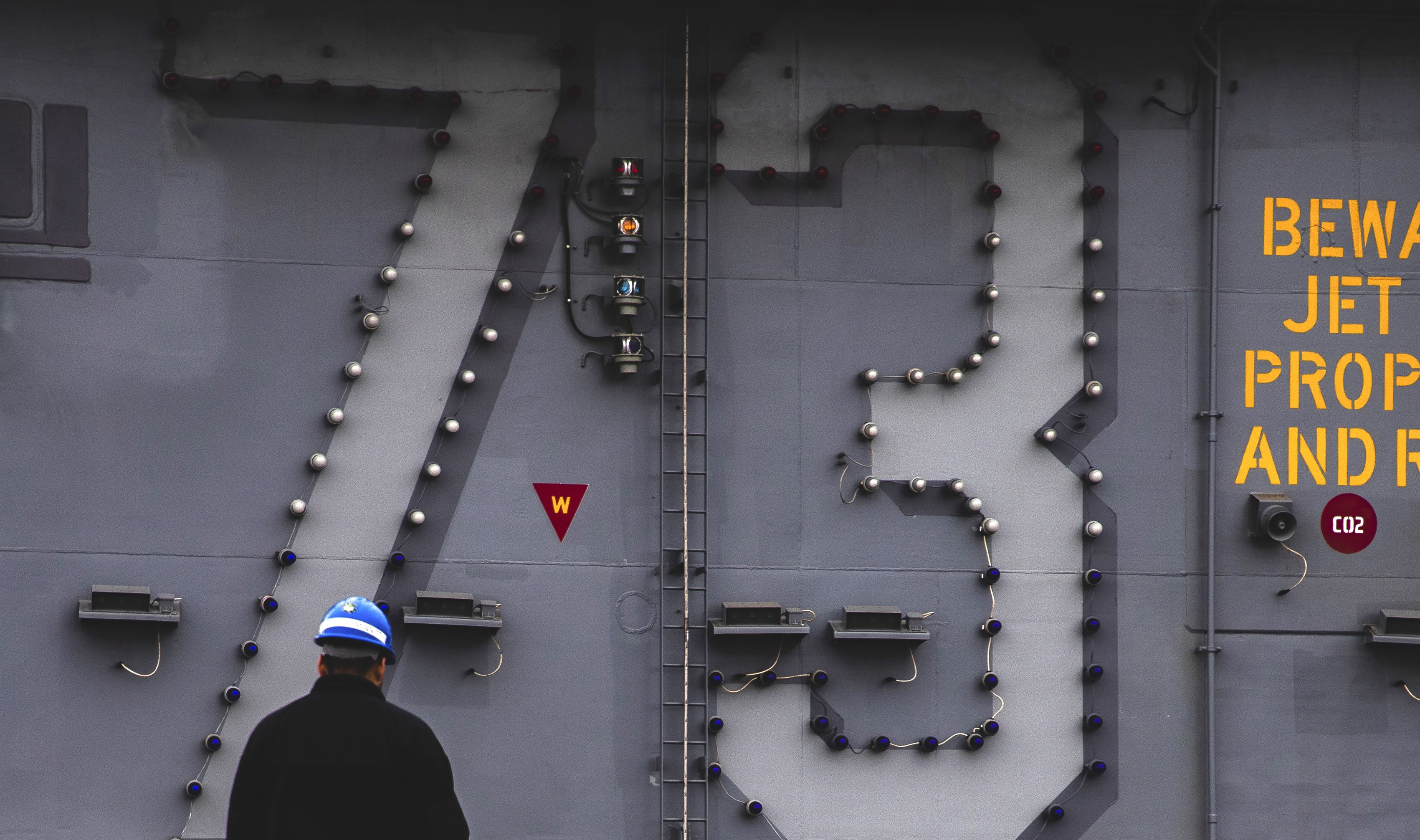This photograph captures the side of a large, gray metallic wall, which could either belong to an industrial site or the hull of a ship, featuring the large white number "73" prominently painted on it. The numbers are outlined with a series of white and black dots, possibly light bulbs or rivets. Next to the "73," several cameras are mounted—in red, yellow, blue, and black—along with a small red circle that reads "CO2". On the right side of the image, partially cut off yellow text reads "BEWARE JET PROP," suggesting the presence of a jet propulsion system. An upside-down red triangle with a yellow 'W' is also visible. Additionally, a ladder is mounted vertically between the '7' and '3', accompanied by siren-like alarm lights. In the bottom left foreground, a man is seen wearing a dark black jacket and a blue helmet with a white stripe, looking away from the camera towards the wall. His face is obscured, focusing directly on the area where "73" is painted.